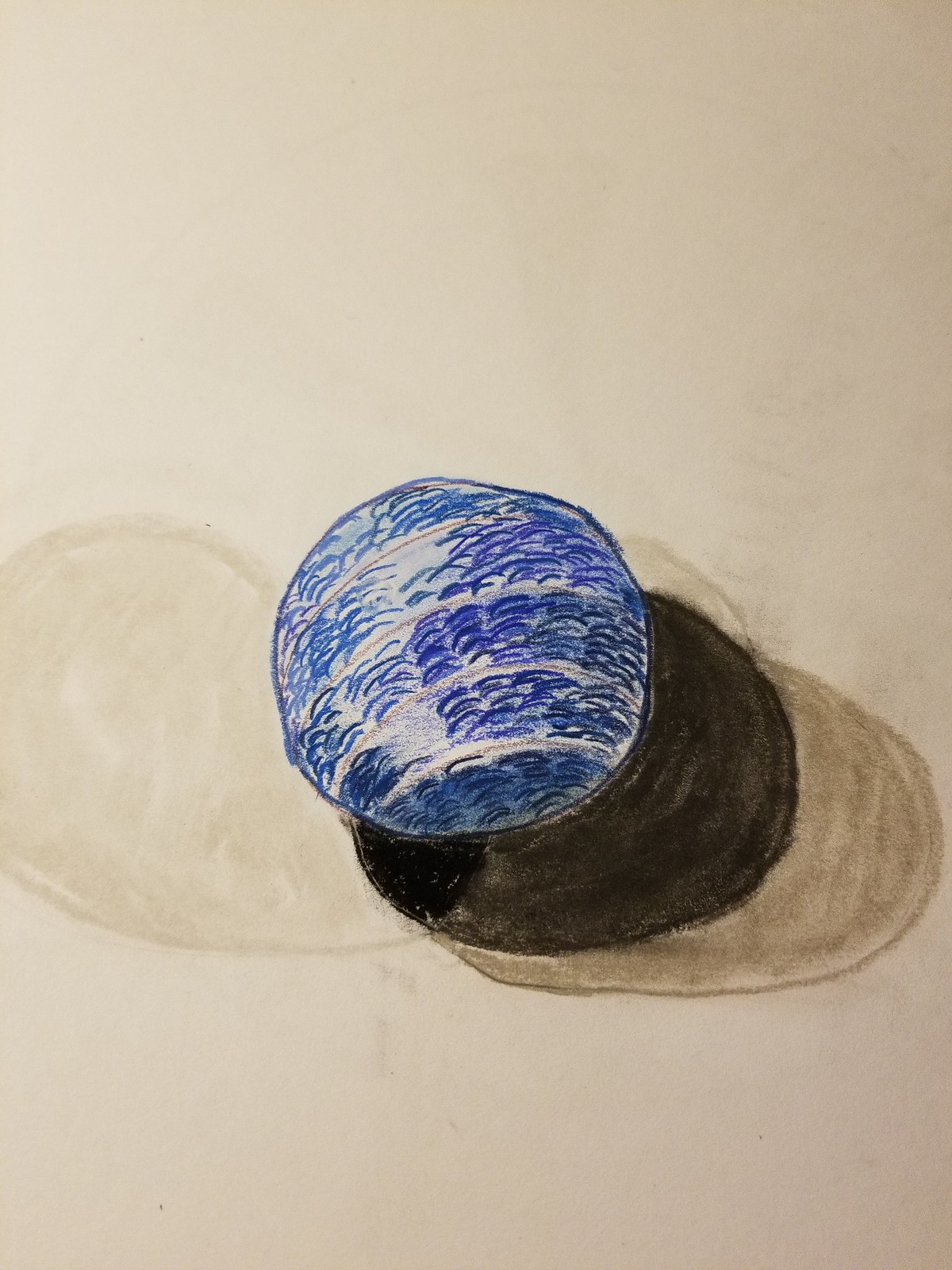The image showcases a unique drawing on an off-white, almost tannish paper. Dominating the center is a blue-shaded circle with rippling white stripes and short black lines, giving it a spherical appearance. To the left, behind this blue circle, is a larger, very pale gray shaded circle. To the right, also behind the blue circle, is a deeply shaded, almost black, crescent shape, which arcs out from under the blue circle. A very light gray shadow extends further to the right of this dark crescent. The shading and coloring appear to utilize a pen or pencil tip, creating varied textures. The juxtaposition of these elements against the off-white background adds depth to the drawing, though the exact nature or purpose of the shapes remains abstract and open to interpretation.